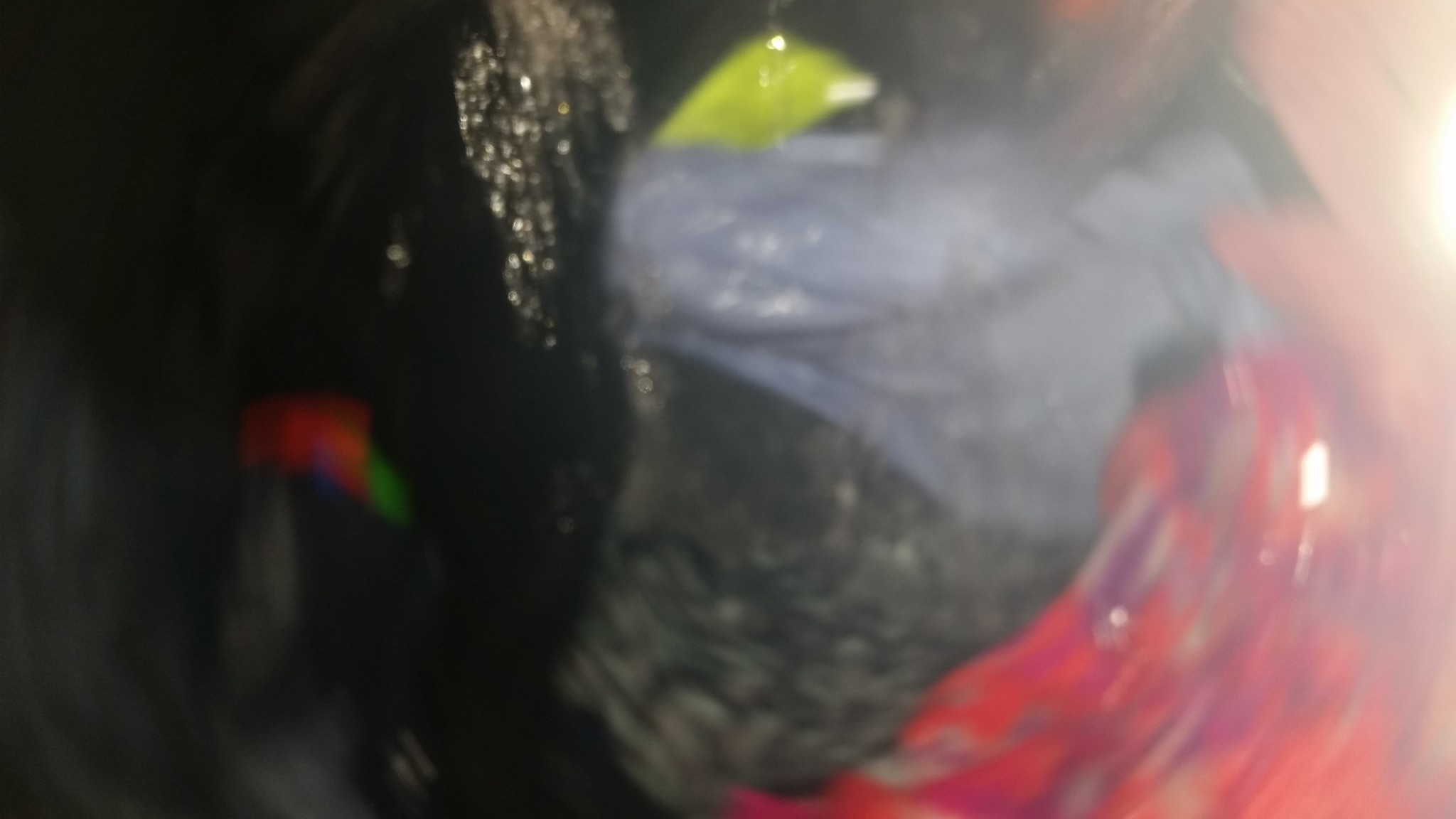The image is a dynamic and heavily blurred action shot, likely capturing the swirling motion of a washing machine in action. It features an array of vibrant, swirling colors—including prominent hues of pink, purple, blue, gray, black, and yellow—giving the overall impression of a chaotic yet colorful whirlpool. Distinct water-like elements are noted, dripping from the top of the image towards the center. In the center, a light blue area contrasts against a darker background, and there are sections resembling a yin-yang symbol with black and very light blue. The left side is predominantly black, while the right side appears smeared, as if the photographer was moving rapidly. The image's composition includes possible shiny, silver parts, adding to the complexity and reflecting light in various directions, enhancing the blurriness. Overall, the photograph is characterized by its colorful, motion-filled pattern, with the swirling and smeared elements making it difficult to discern specific objects within the scene.